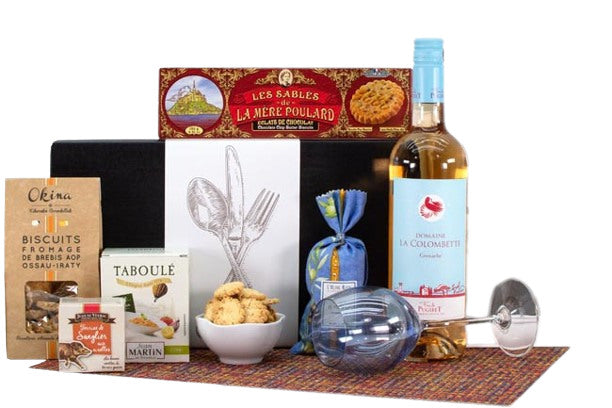The image presents an elegantly arranged picnic scene on a colorful, possibly knitted, mat beside a serene pond. Dominating the right section of the image is a horizontally placed wine glass, adjacent to a standing bottle of white wine with a distinctive blue cap and a label reading "La Colombetti." Next to the bottle, a blue bag possibly holding biscuits is situated near a white bowl filled with yellowish croutons or biscuits. Moving leftwards, a white cardboard box inscribed with "Taboo" is partially obscured by a smaller container adorned with a pig illustration. On the far left, a cardboard container mentions "Biscuits from March." Behind all these items, a black rectangular box, featuring a white logo with a spoon, fork, and knife, supports a red box labeled "Lame Pollard," displaying biscuit and castle images. The diverse assortment of at least five or six different packaged biscuits, some in boxes and others in paper bags, along with the bowl of biscuits, exudes the essence of a luxurious French picnic spread.